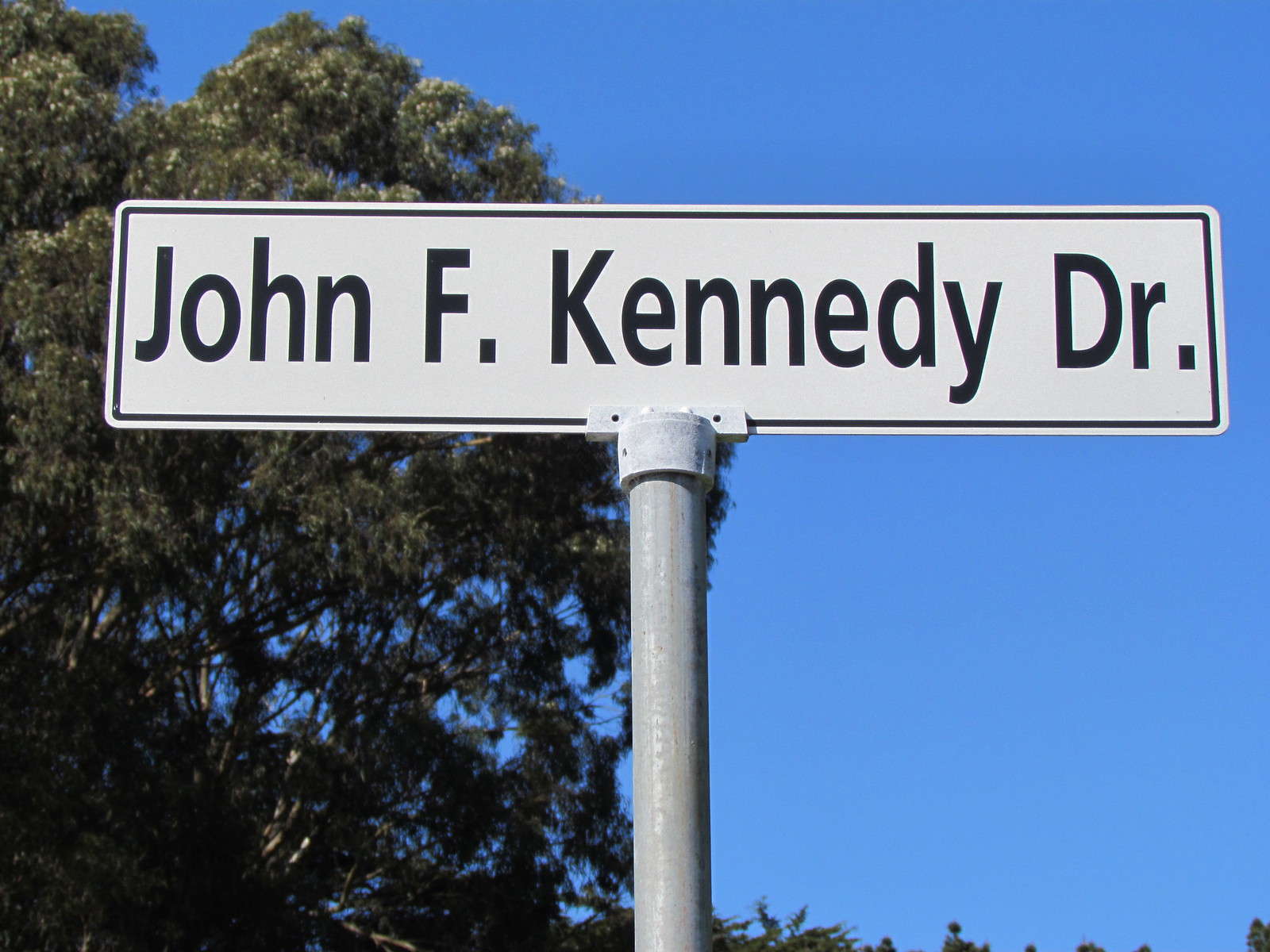This square-shaped outdoor image showcases a clear blue sky in the background, accompanied by lush green trees on the left side and tree leaves at the bottom. Central to the image is a gray, round pole supporting a rectangular white sign with a black border. The sign's bold black text reads "John F. Kennedy, D.R."